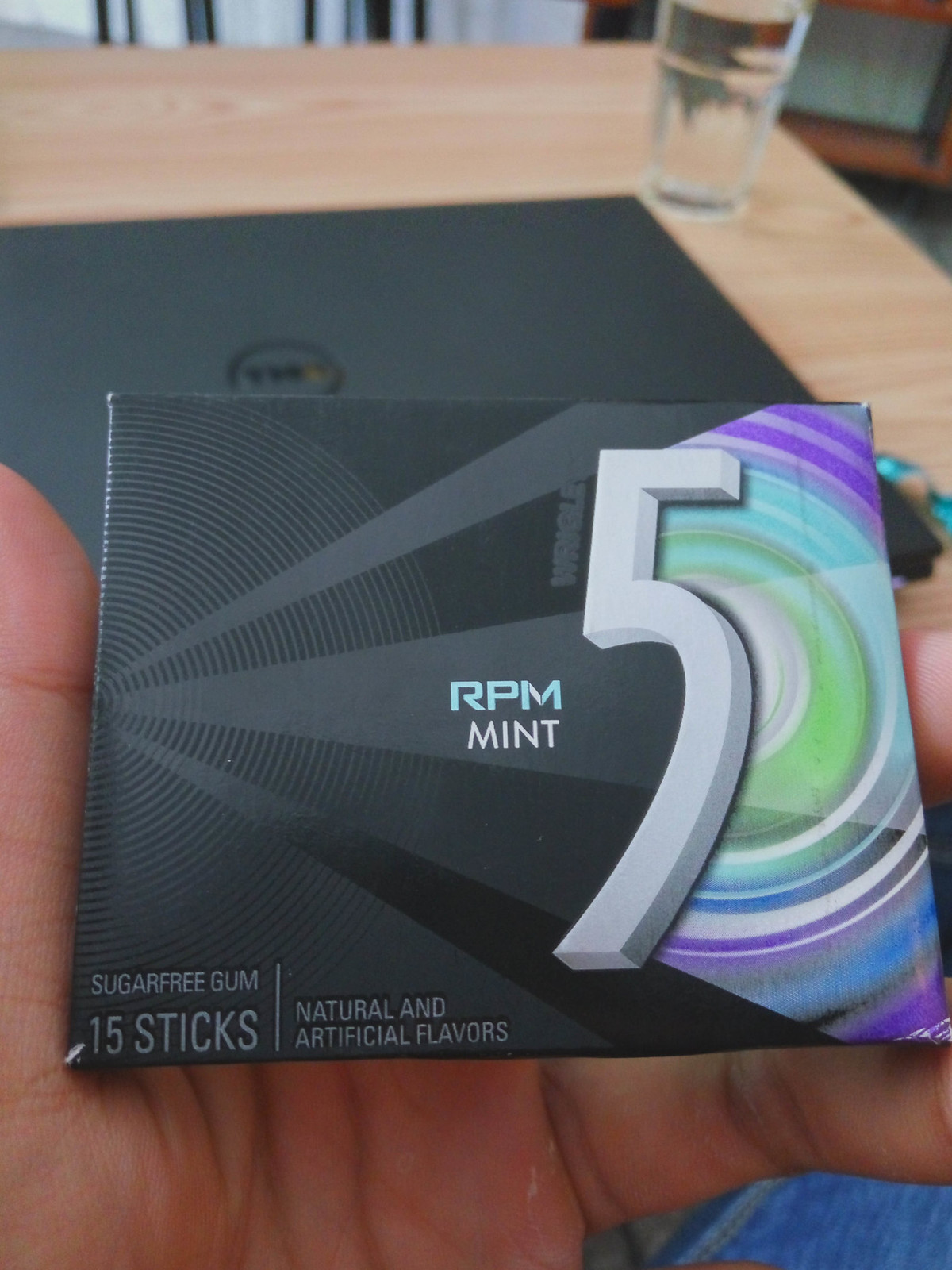The photograph presents a close-up of a stylish, square pack of RPM Mint chewing gum held by a Caucasian individual with their left hand, with the gum pack pinched between their thumb and middle finger. The packaging is predominantly black with a striking design that includes a futuristic sunburst pattern radiating from the background. A prominent white number "5" adorns the right side of the pack, surrounded by colorful concentric half-circles in shades of green, white, blue, and purple. The gum's name, "RPM Mint," is displayed boldly in green and white at the center, indicating the flavor. The text on the bottom left of the pack states "sugar-free gum, 15 sticks, natural and artificial flavors." The scene is set on a light wooden table, with a laptop closed in the background to the left and a glass of water positioned in the upper right corner, complementing the relaxed and casual ambiance.